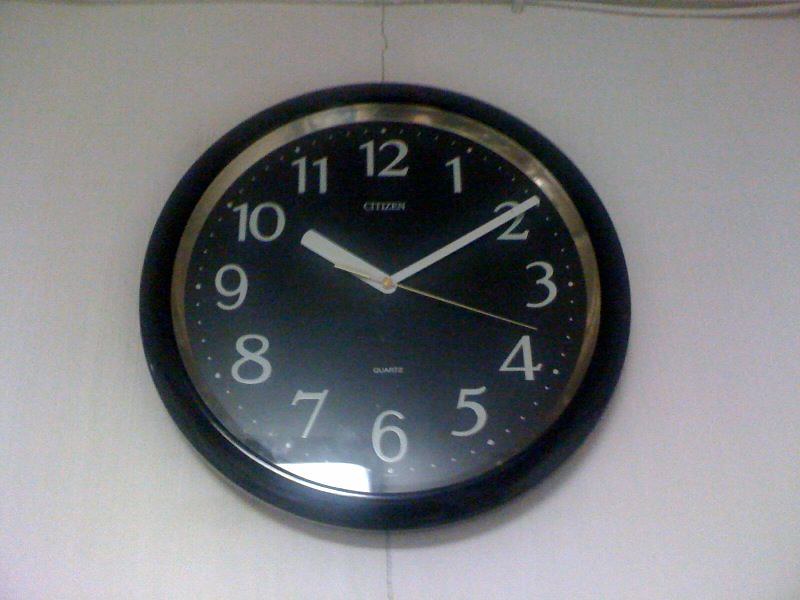In this detailed photograph, we see a circular wall clock prominently mounted on a white wall. The clock features a sleek black plastic frame, encircling a subtle gold bevel that adds a touch of elegance to its design. Within the gold border, the clock face is black, contrasted by white numerals in a standard font, marking every hour from 1 to 12. There are small white dots between each number, denoting the minutes. At the top of the clock, just below the 12, the brand "Citizen" is clearly visible, while at the bottom, above the 6, the word "Quartz" is inscribed. The hour and minute hands, both white, indicate the time as 10 minutes past 10, with a slender yellow second hand ticking steadily. This classic design, with its clean black, white, and gold palette, offers a timeless and understated elegance.